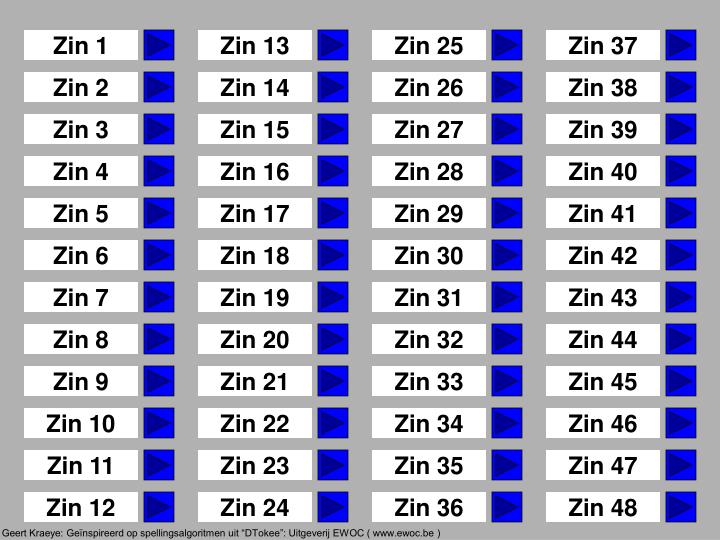The image features a detailed table set against a gray background, consisting of 48 white labels arranged in four columns and 12 rows. Each label is a white rectangle with adjacent dark blue squares containing right-pointing arrows. The labels are sequentially numbered from "ZIN 1" to "ZIN 48," written in a black, Times Roman font. The sequence starts in the top left corner with "ZIN 1" and continues down each column, finishing in the bottom right corner with "ZIN 48." At the bottom left of the image, in small black text, there is a collection of foreign words and abbreviations, including "GERTKRYE," "GIN SPI REE RD," "OP," "ALGO N T L M E N," and "UIT." Additionally, it mentions "DTOKEE" in parentheses with a web address "www.ewoc.be" also in parentheses. The foreign text appears to be German.